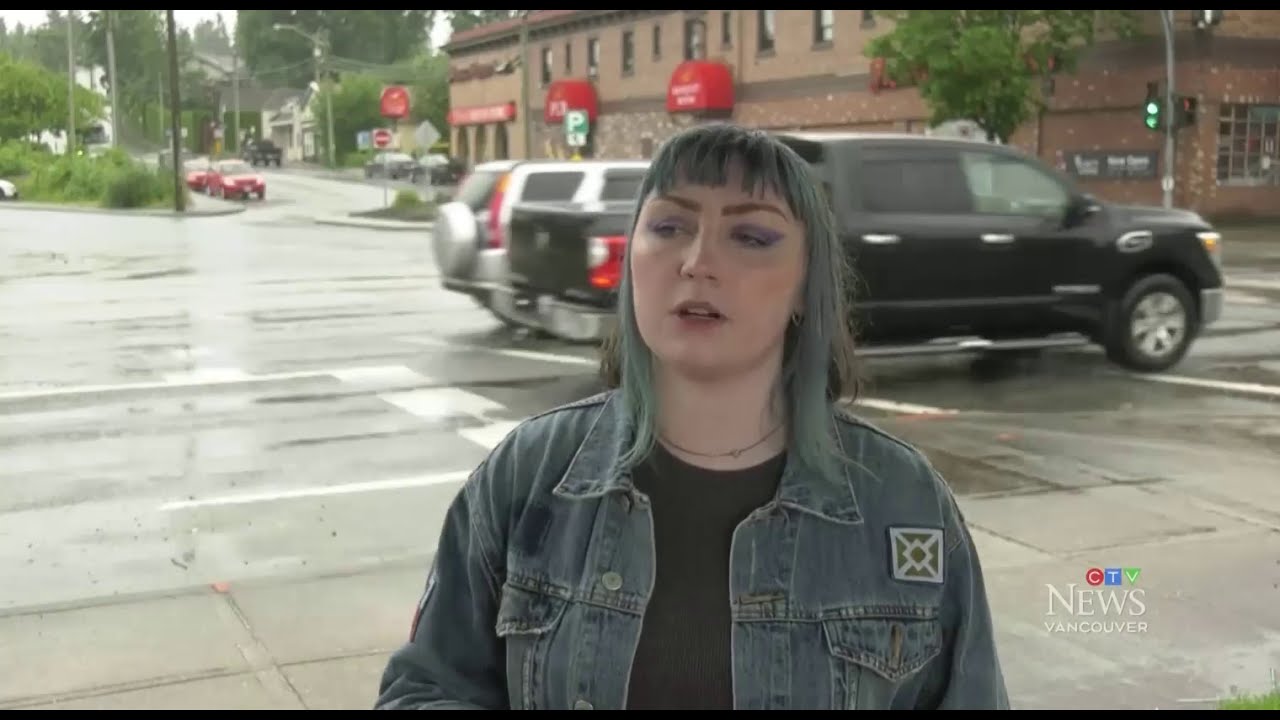In the image, a woman who appears to be in her early to mid-30s stands on a sidewalk near a busy intersection, identifiable by the CTB News Vancouver logo in the bottom right corner. She has distinct bluish-green hair with very short-cut bangs and wears tiny gold hoop earrings. Her makeup features gray eye shadow that extends to pointed corners, adding a slightly gothic touch. She has light skin and brownish, obviously drawn-on eyebrows. 

She is dressed in a gray denim jacket with a black undershirt, and her jacket has pockets and a unique insignia featuring a diamond-shaped X inside a square. A form-fitted chain necklace adorns her neck. She is looking off to her right, and the image captures her from the chest up.

In the background, a black pickup truck and an SUV are traveling along the road. On the opposite side of the road, there's a brown building with two red awnings that appears to be a shop, while a green traffic light is visible near this building. The scene also includes a commercial parking lot further back, along with hints of a residential area in the distance.